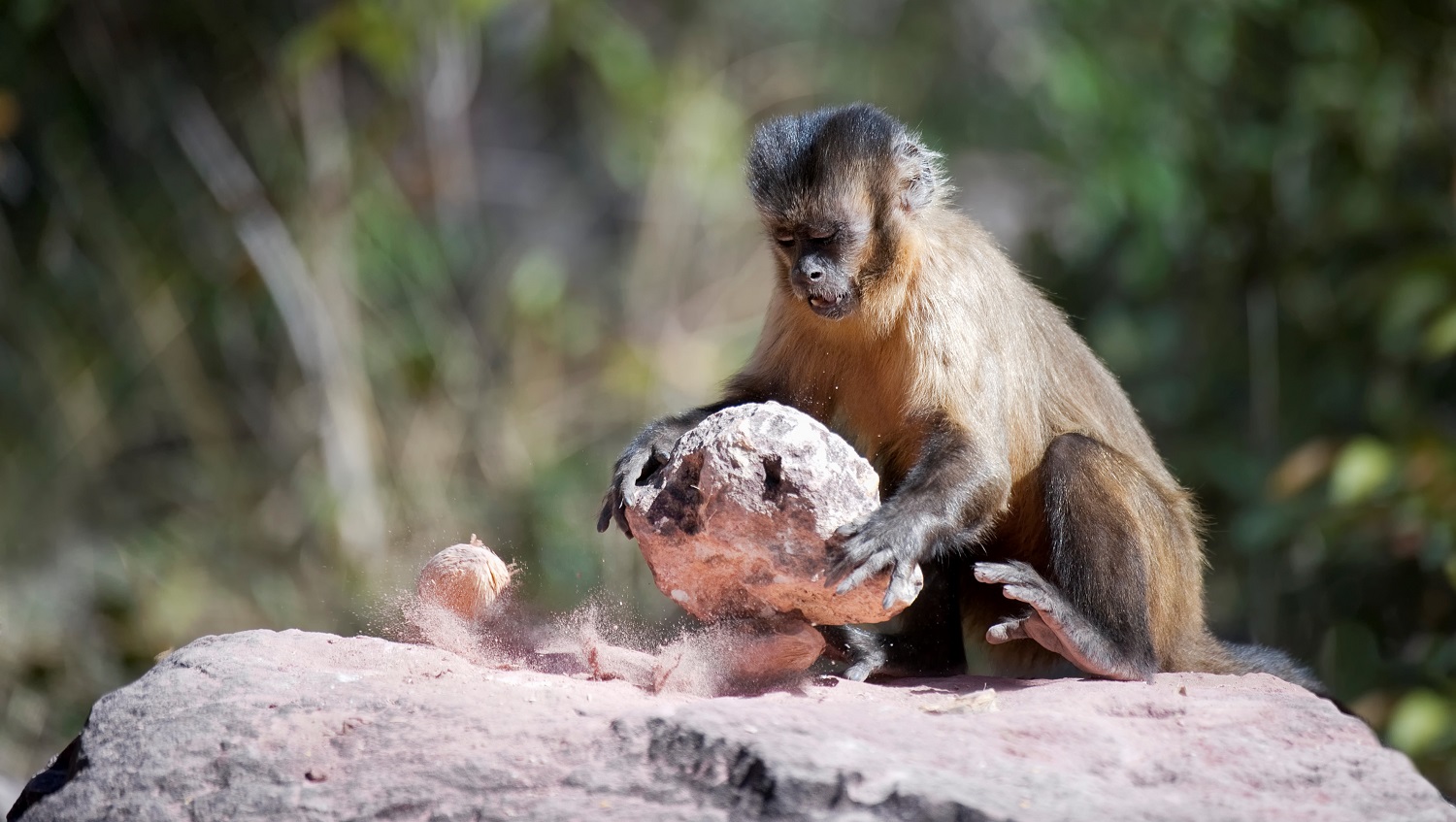In this detailed outdoor photograph, a light brown monkey with a darker patch on the top of its head is the clear focal point. Sitting atop a larger boulder, the monkey is in focus, with its concentrated gaze directed downward as it uses a large stone as a tool to break open a coconut. Bits of the coconut are scattered around the boulder, showcasing the monkey's determination and precise effort. The background features blurred trees illuminated by sunlight, casting a warm glow on the monkey's back and enhancing the scene's natural charm.